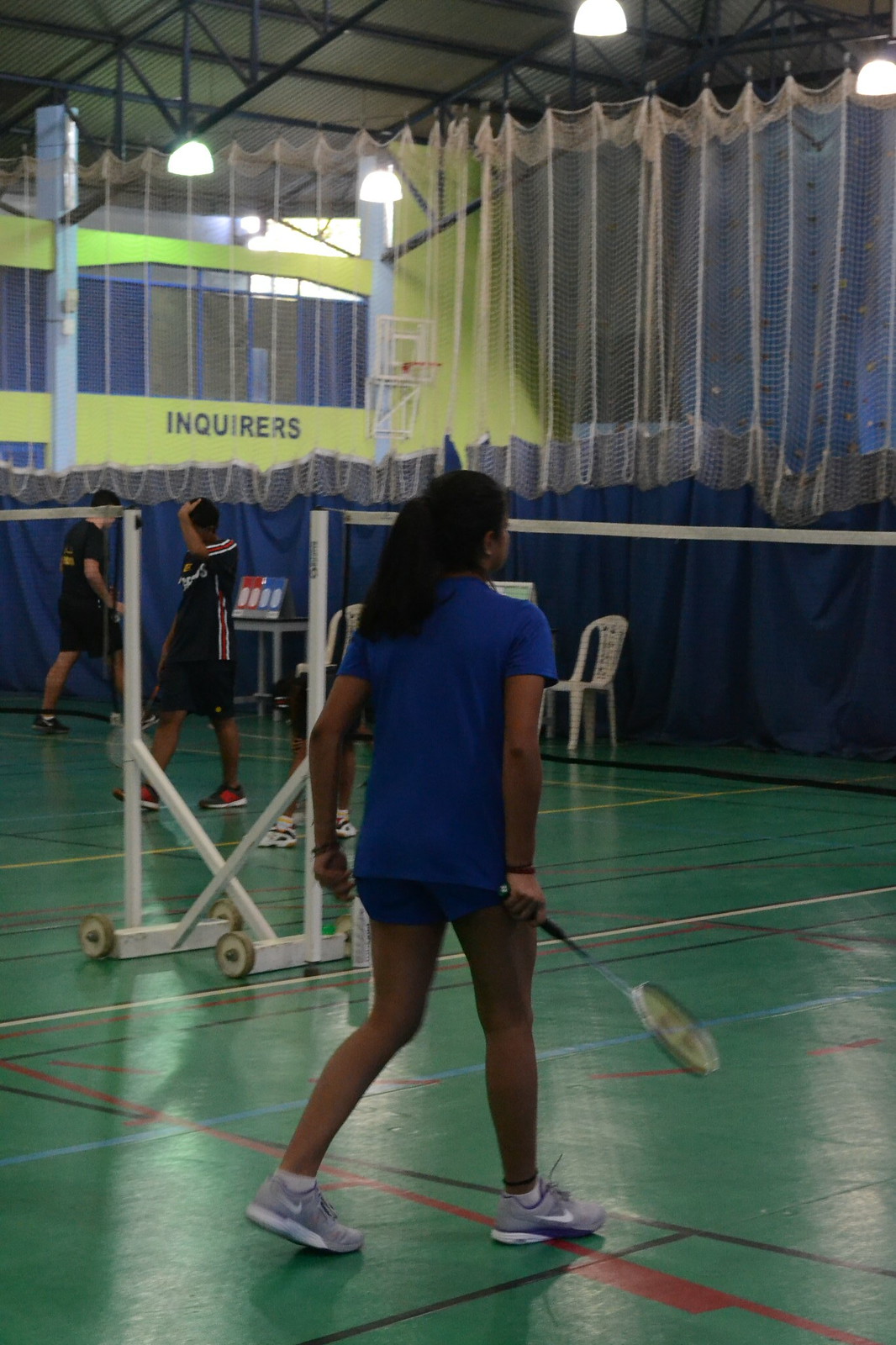In this detailed photograph of an indoor gymnasium, two parallel badminton courts can be seen, each marked with an array of colorful lines—red, light blue, white, yellow, and black—on a green floor. Separating the two courts is a blue cloth and white netted divider. Both nets are mounted on wheeled white structures that appear somewhat temporary and not particularly sturdy.

At the center of the image stands a female player with her back to the camera. She is positioned toward the right side of the court, poised and seemingly ready to return a shuttlecock. Her long black hair is tied back into a ponytail, and she sports a matching blue outfit consisting of a short-sleeve t-shirt and shorts. On her feet are gray Nike tennis shoes, distinguished by their white swooshes. In her right hand, she holds a thin badminton racket.

To her left, on the adjacent court, two male players in dark navy blue uniforms are engaged in their own game. One of them appears to be expressing frustration, possibly having just made an error. The net on their court stretches across the width of the gym, which is characterized by its high ceiling and expansive, multifunctional design, as indicated by the multiple lines and temporary net structures.